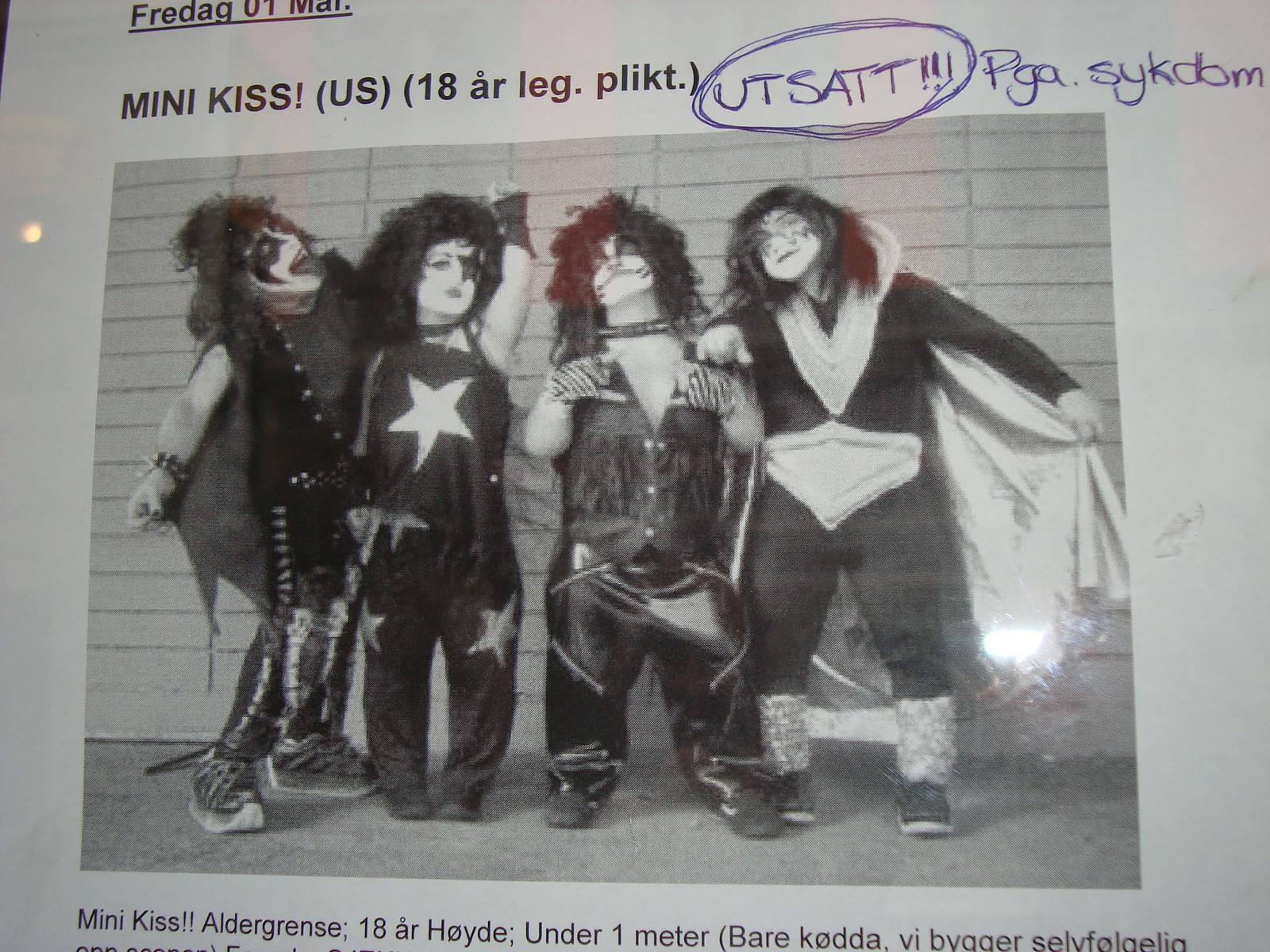This black and white photo captures a promotional poster for a band called "Mini KISS," a tribute band where all members are under one meter tall. Positioned at the top left, the text reads "FEDAG U1MAL," followed by "MINIKISS US18AR LEGDOT PLICT." Prominently handwritten in blue ink and circled for emphasis is "UTSATT! PGA SYKDOM," indicating a cancellation due to illness. The bottom of the poster features a striking image of four musicians dressed in full KISS regalia, complete with iconic KISS makeup, black leather outfits, and dramatic capes. Each band member captures the essence of KISS with their attention to detail, including one member sticking out his tongue, reminiscent of Gene Simmons. The text further emphasizes their unique attribute by noting that all members are under one meter tall. The overall composition of the poster marries rock and roll nostalgia with a playful twist, capturing the essence of the "Mini KISS" experience.